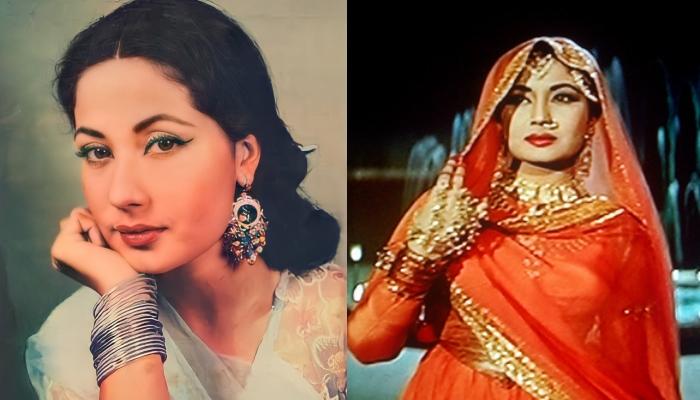The image displays two distinct photographs of an Indian woman, possibly the same individual in different settings. The photograph on the left captures a close-up of the woman in a sitting position, with her head propped on her right hand. Her large, intricate earrings featuring colorful stones like blue, white, and yellow dangle prominently. She wears a bracelet with numerous small silver rings on her wrist, and her hair is neatly slicked back in an updo. Dressed in a white outfit, she engages viewers with a direct gaze. The photograph on the right showcases the woman standing in an elaborate orange-red dress with a diagonal gold strap. Accessorized with plentiful jewelry, including a handpiece that wraps around her fingers and wrist, and a possible nose piercing, she stands with a water fountain in the background. Her red veil adds a touch of cinematic flair, reminiscent of a Bollywood scene, as she looks slightly to her left, her red lipstick complementing the traditional attire.